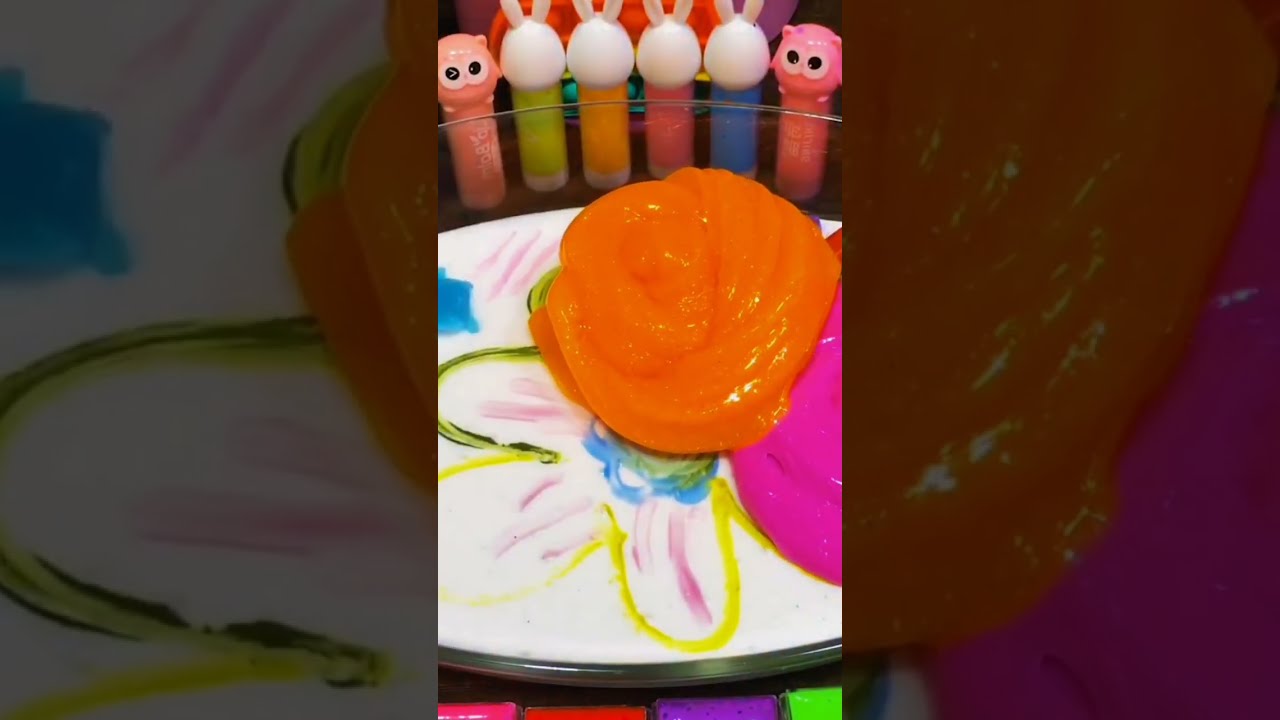The image features a vividly colorful scene centered around a white plate with black accents, adorned with intricate blue flowers that have yellow petals and blue and green centers. On the plate, there is a shiny, almost circular glob of orange goo, as well as a few spots of bright pink goo. The plate rests on a vibrant surface splashed with shades of pink, red, purple, and green. In the background, there is a clear tray holding six sticks, with each end stick topped with a cute cartoon animal face, while the middle four merely have white circular caps. Additionally, the background appears blurred and is dotted with neon-colored bottles resembling cartoon characters, including owls and rabbits, in hues such as light pink, neon green, neon orange, bright pink, and neon blue. The image has a rectangular layout with blurred and magnified borders that echo the colorful splatter and vibrant tones of the main scene, enhancing the whimsical and playful atmosphere.